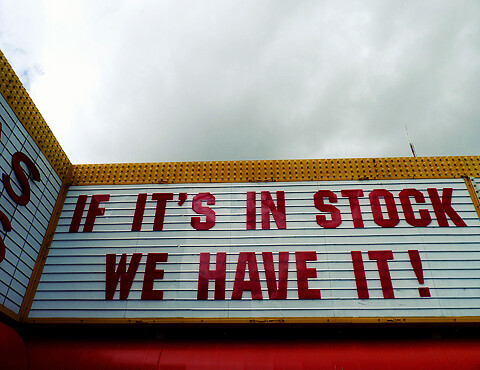This photograph, taken outdoors from a low angle looking upward, captures a marquee sign against a sky covered with white and gray clouds. A faint bit of blue sky is visible at the top left corner, while darker gray clouds dominate the top right. The marquee sign, reminiscent of an open book, extends from the left to the right, adorned with a textured, studded gold trim. The left side of the sign features a partial white section with a red letter "S," framed by a brownish-gold border. The right side presents a clear message in red letters: "IF ITS IN STOCK, WE HAVE IT!" Beneath the sign is a red wall, casting a black shadow, further emphasizing the sign's prominence against the cloudy backdrop.